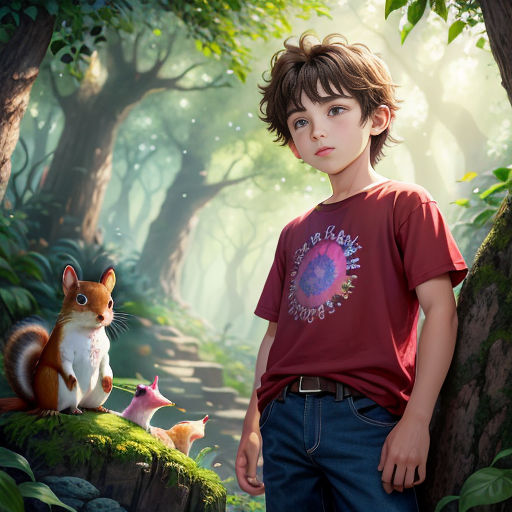In this animated image, a Caucasian boy with somewhat curly brown hair, parted to the side, stands in a mystical, overgrown forest. He is wearing a maroon-red shirt adorned with a peculiar design featuring a pink circle and purple accents in the middle, partially tucked into his blue jeans, revealing a brown belt with a silver buckle. His arms rest comfortably at his sides. To his left, there is a sizable orange squirrel with a white underbelly, looking directly at him. On a mossy rock next to the squirrel, there are vivid pink and orange slugs. The forest around him is dense with large trees bearing green leaves and brown trunks, their blurred forms creating a dreamy backdrop. Rays of daylight penetrate through the foliage, adding an enchanting, almost magical light to the scene. The forest floor is dotted with grass and remnants of what appear to be old, crumbling bricks, suggesting the area was once different before nature reclaimed it.